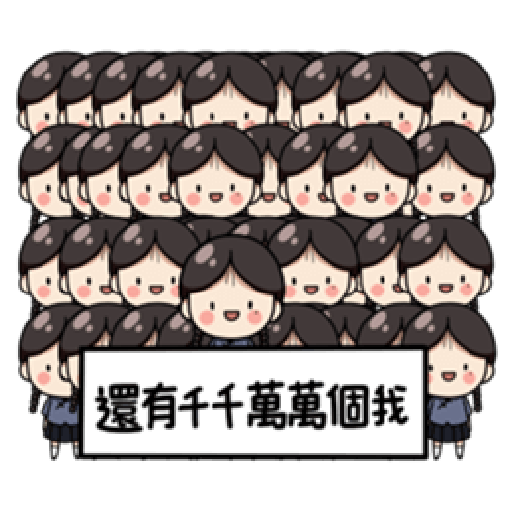The image is a detailed drawing of rows of animated Chinese girls, organized into four rows, each containing around 9 to 10 girls. All the girls share identical features including a middle-part hairstyle with bangs swooping down and tucked behind their ears. They have tiny, dark brown eyes, small pink noses, and round pink cheeks, giving them a lively appearance. Their reddish mouths are outlined in black, with a flat top and a semi-circular bottom, suggesting a subtle smile. Each girl is dressed in a blue-purple shirt, a black skirt, and white socks. A notable detail is the illumination on the left side of their dark brown hair, appearing slightly lighter. In the bottom row, one girl's head sticks up and out, drawing attention. This row also features a body holding up a white banner with Chinese text in black symbols, contrasting against the uniformity of the group's animated heads.